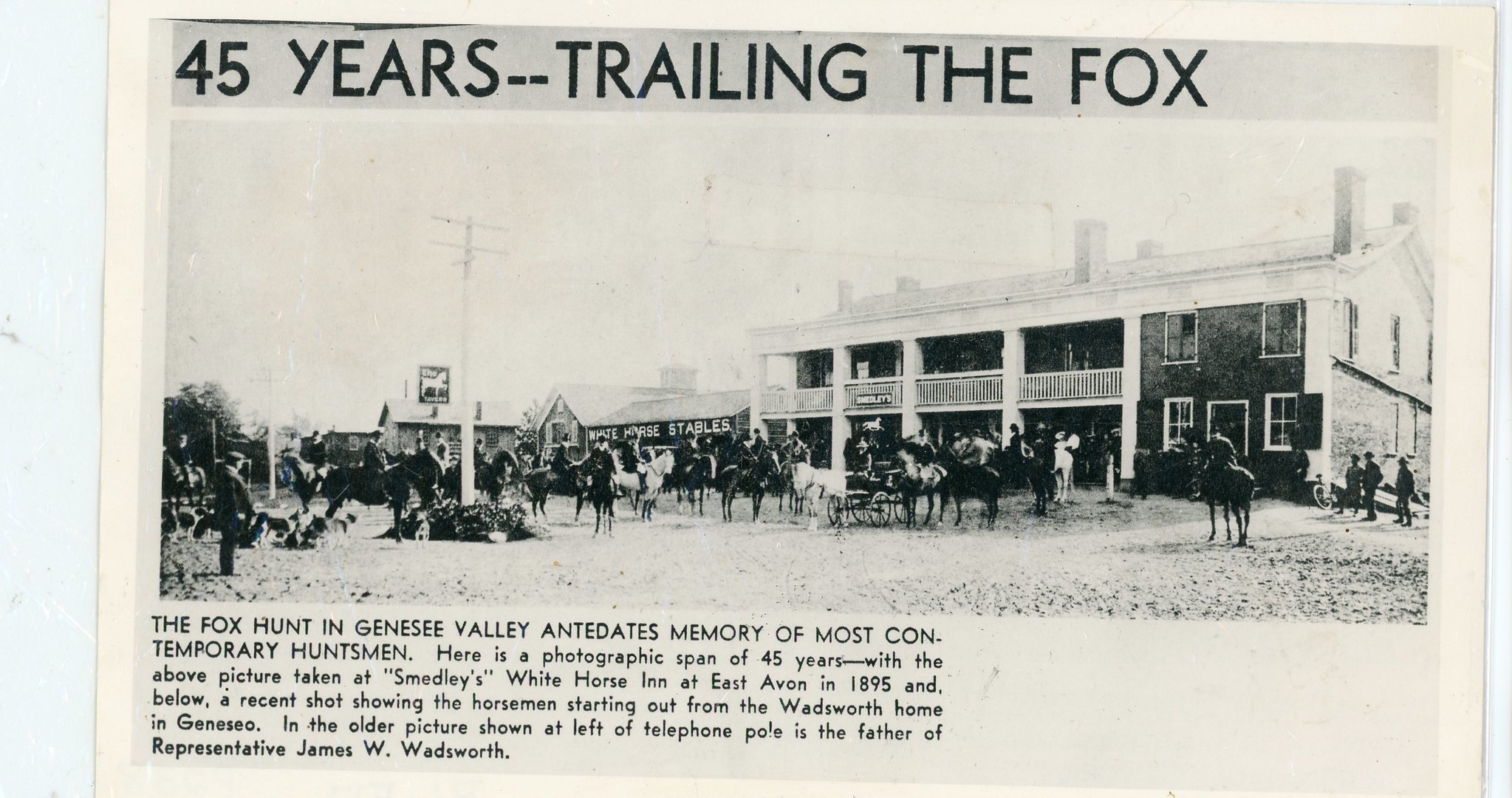The image is a photograph or scan of an antique newspaper or publication page, slightly yellowing with age. At the top, in a gray box, the headline reads "45 YEARS TRAILING THE FOX" in capital black letters. Beneath this, a large black-and-white photograph depicts a scene of several dozen people on horseback gathered in front of a notable two-story building with white posts and a white roof, identified as Smedley's White Horse Inn in East Avon. The photograph captures a historic moment from 1895, just before a fox hunt. To the right of the image, a telephone pole is visible, and to its left stands the father of Representative James W. Wadsworth. At the bottom left of the image, the bolded capitalized caption reads: "THE FOX HUNT IN GENESEE VALLEY ANTEDATES MEMORY OF MOST CONTEMPORARY HUNTSMEN." In smaller, unbolded letters, it provides a contrast with a recent photograph showing horsemen departing from the Wadsworth home in Geneseo, emphasizing a 45-year photographic span. The scene includes not only horsemen but also a man in a buggy and a few men on foot, enhancing the depiction of a vibrant moment from a bygone era.